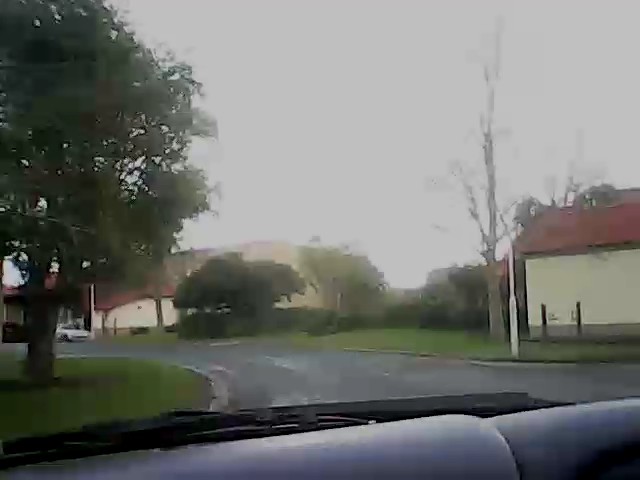In this image of a residential area, a long black driveway guides the eye into the scene. A large, lush tree stands prominently in a grassy area, which is encircled by a concrete barrier. To the right, another tall tree reaches skyward, its branches mostly bare save for a few scattered leaves. An off-white building with a red roof sits to the side, complementing the surrounding scene. In the foreground, there is another building with a tan exterior, positioned next to a similarly off-white building with a red roof. A white car is parked in front of these structures, enhancing the everyday charm of the neighborhood setting.